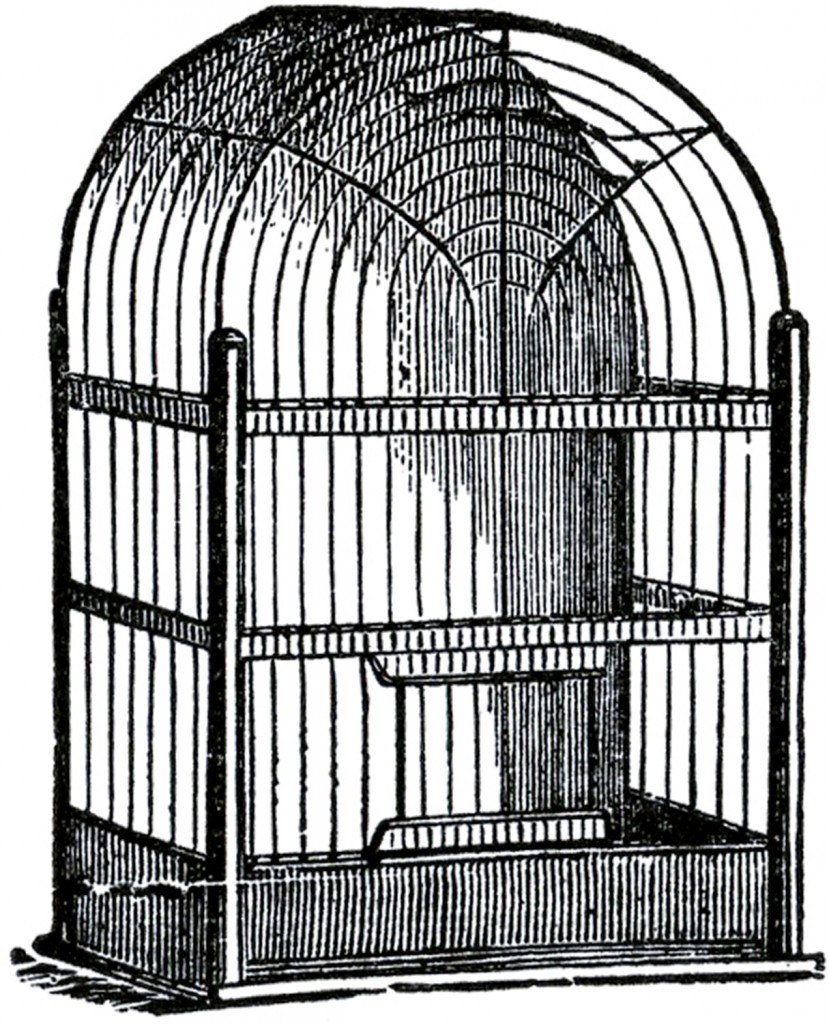This detailed illustration, rendered in black-and-white pen-and-ink style, depicts a vintage birdcage with a prismatic base and a rounded top. It features a solid base supported by four posts, each segment intricately shaded and textured, giving it a realistic, hand-drawn quality akin to reproductions from old magazines or manuals. The cage is depicted with multiple levels or layers, crossbars, and what appears to be a door at the front center, slightly tilted to the viewer's right. Despite its apparent design and structure as a birdcage, it notably lacks any birds, perches, or other entities inside or outside, emphasizing its presence as an elegantly detailed container on a pristine white background.